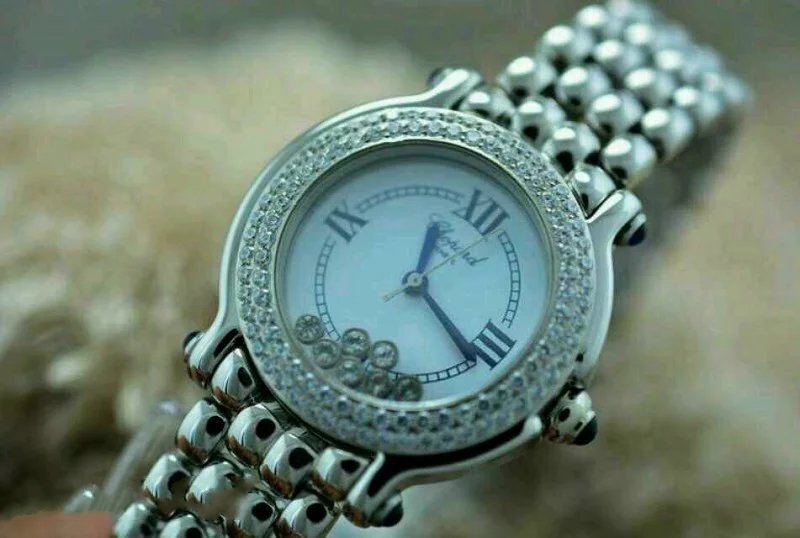A detailed close-up view of a luxury lady's watch is depicted. The watch is angled almost completely to the right, with the top of the band facing the top right corner and the bottom of the band positioned near the center left of the image. The watch band is crafted from tightly placed silver beads.

The watch's outer face is adorned with two rows of very small diamonds. The watch face itself features a pristine white background and displays Roman numerals at the 12, 3, 6, and 9 o'clock positions. The hour and minute hands are black, while the second hand is a striking gold. Towards the bottom of the watch face, there are seven loose diamonds, which add an extra touch of elegance.

Under the 12 o'clock position, the brand name "Chopard" is inscribed in cursive writing. The winder, located on the right side, is silver with a rounded black top. Both the top and bottom connections of the watch face to the band feature a raised silver design with rounded black tops, matching the winder.